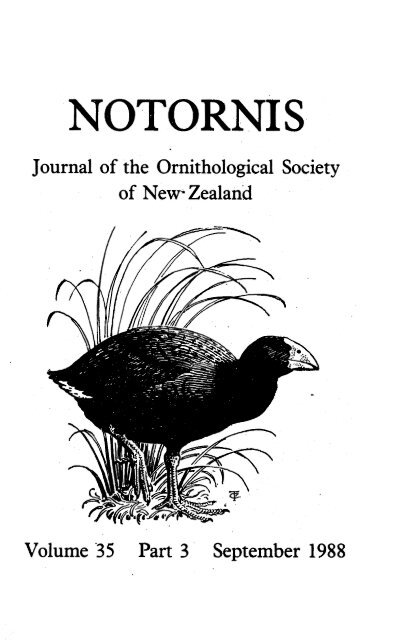This black and white image features the cover of the "Notornis, Journal of the Ornithological Society of New Zealand," prominently displayed in bold capital letters at the top. Below the title, the subtitle reads: "Journal of the Ornithological Society of New Zealand." Centrally positioned on the cover is an artistic black and white drawing of a bird standing amidst tall grass. The bird, characterized by a fat abdomen and a wide beak, is depicted mid-step with one foot on the ground and the other raised. The detailed depiction includes the bird’s talons and shading that suggests a dark coloration, though the exact color cannot be discerned due to the monochromatic scheme of the image. The grass surrounding the bird is rendered in a mix of black and white tones, complementing the overall aesthetic. At the bottom of the cover, the publication details are clearly stated: "Volume 35, Part 3, September 1988," distributed across the lower portion in an organized manner with black text against a contrasting white background.